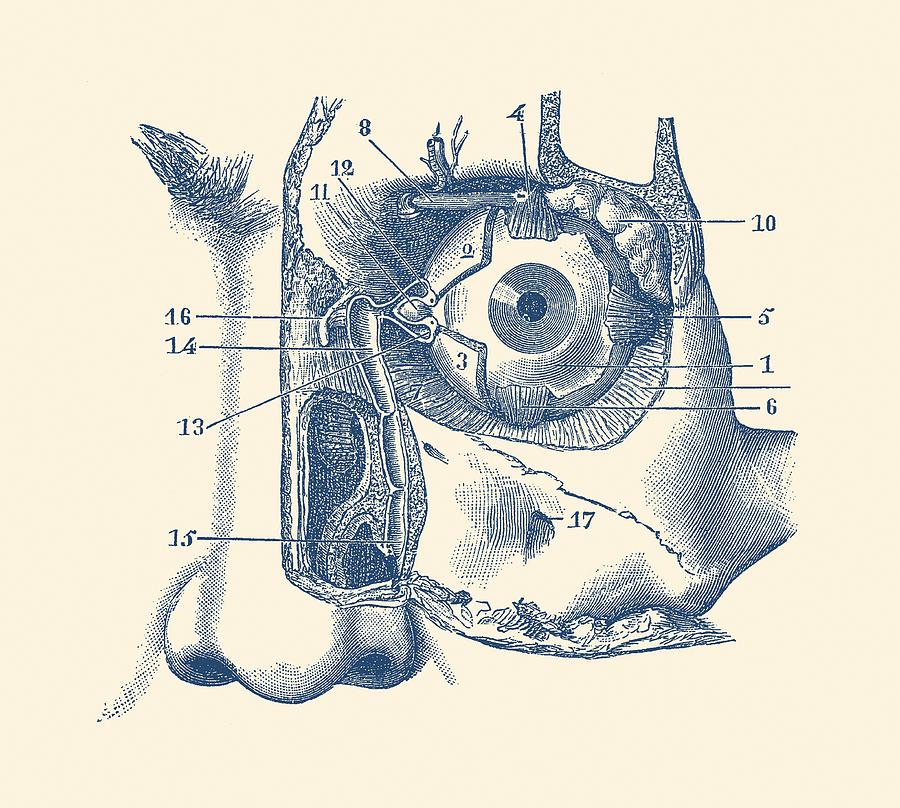This is a detailed, black-and-white, vintage scientific illustration, likely from an old textbook, depicting the anatomy of the human eye along with partial views of the nasal area and cheekbone. The left side of the illustration reveals parts of the nose, while the right side focuses on a single eye within the facial structure. The intricate drawing has the skin peeled back to expose the underlying layers, showcasing the full eyeball, various muscle structures, and other internal components. Each area of interest is meticulously labeled with numbers from 1 to 17. For instance, number 1 marks the eyeball itself, and number 10 identifies the eyelid fat beneath the skin. This ink-drawn and printed illustration highlights detailed anatomy through its numbered sections, clearly pointing to the iris, eye muscles, and various other parts, making it an educational resource rich in detail and precision.